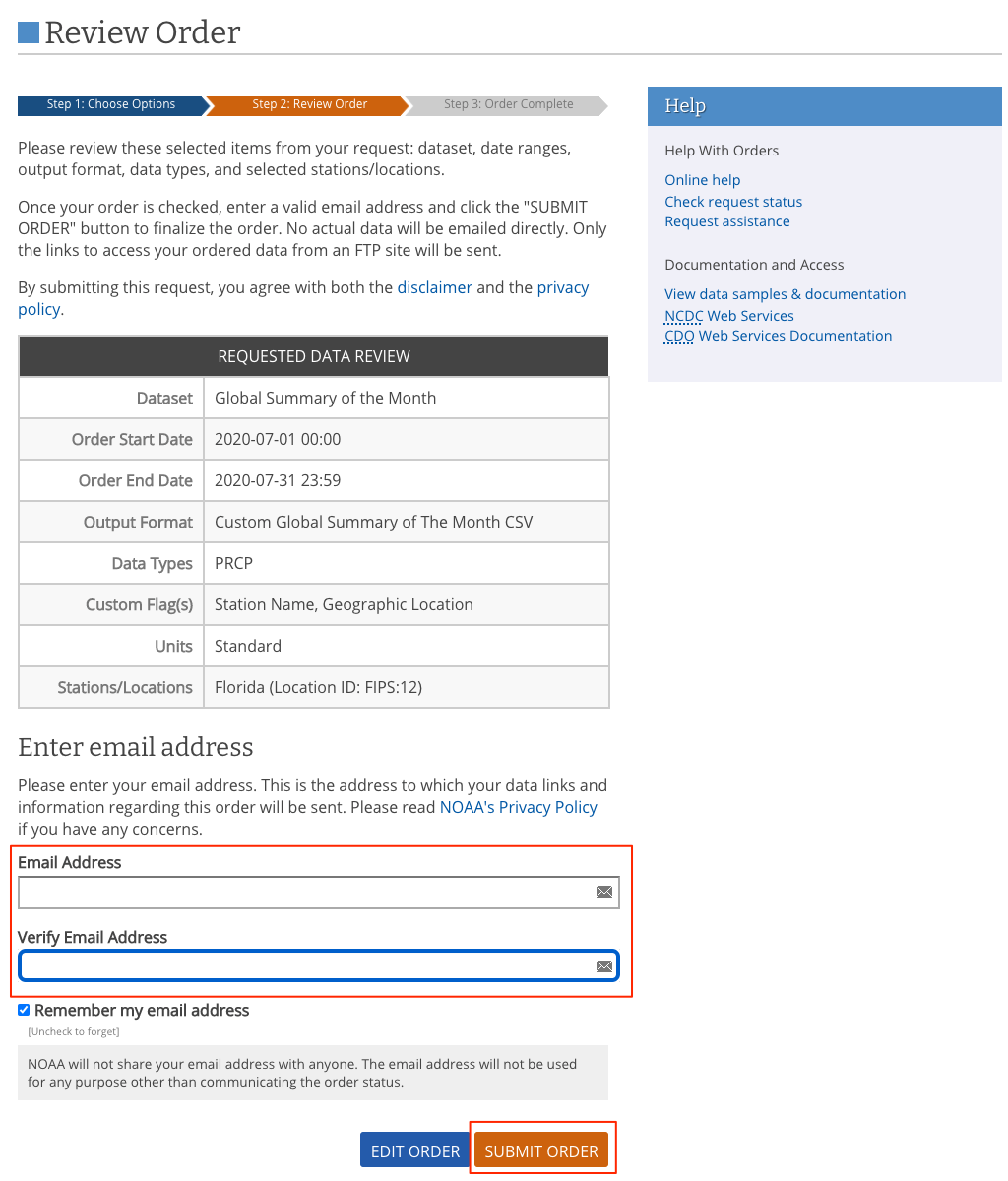Screenshot of an order review page with detailed directions highlighted:

At the top of the screenshot, there's a white background with a small blue square icon. To the right of this icon, the words "Review Order" are prominently displayed in large, gray letters. Below this title, a thin gray line spans the width of the screen, providing a visual divider.

On the left side under this line, the order steps are illustrated in a sequence of arrows. "Step 1" is inside a blue arrow, "Step 2" is inside an orange arrow, and "Step 3" is inside a gray arrow, clearly indicating the step-by-step progression.

Beneath the step indicators, a message prompts users to "Please review these selected items from your request." Following this is a box labeled "Request a Data Review," which contains detailed information about the review process.

Further down, there's a section to enter an email address. Accompanying the email entry field is a note explaining the necessity for this information. Both the "Email Address" and "Verify Email Address" boxes are highlighted with a red rectangle to draw attention. This red rectangle appears to be an annotation added to guide the user.

At the bottom right of the screenshot is an orange "Submit Order" button, also highlighted with a red box. This final annotation directs users to enter their email address, verify it, and then click on the "Submit Order" button to complete the task.